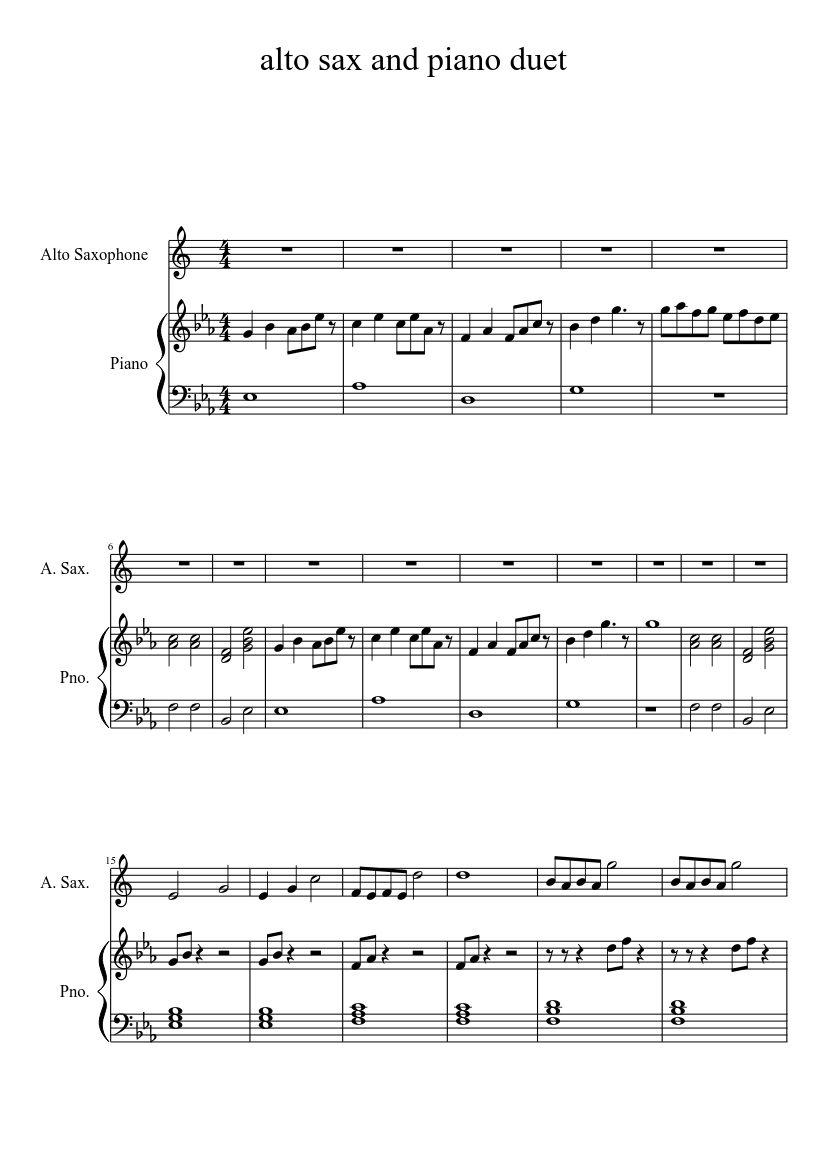The image depicts sheet music for an "Alto Sax and Piano Duet." The music is organized into three sections, each featuring a combination of alto saxophone and piano lines. At the top, the title is prominently displayed, "Alto Sax and Piano Duet." Each section consists of three staff lines: the top line dedicated to the alto saxophone and the bottom two lines grouped for the piano. Notably, the top line abbreviates "alto saxophone" as "A. Sax," and "piano" as "Pno" in the subsequent sections. The composition is set in a 4-4 time signature. The alto saxophone rests for the first few bars and begins playing only in the last row. The entire image is in black and white, featuring all the typical musical notations, including those that resemble golf clubs and other standard music symbols.